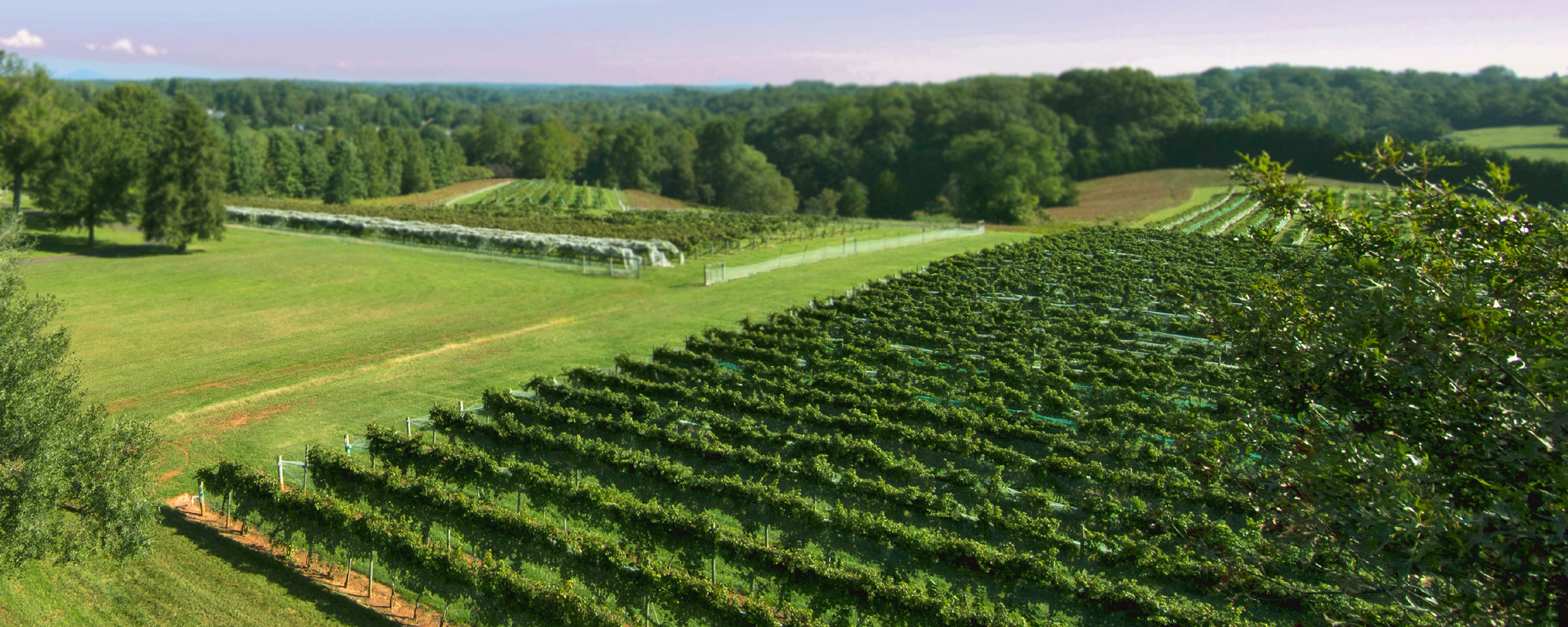This aerial photograph captures a sprawling vineyard, taken from approximately 40 to 50 feet above ground. The sky, beautifully tinged with pink and purple hues, has a few scattered, fluffy clouds, adding to the serene ambiance. Below, neat rows of grapevines stretch out meticulously towards the distant valley, separated by grass strips, giving the appearance of a well-maintained vineyard. The landscape transitions into green fields and is bordered by an expanse of trees. These trees frame the edges of the image, with individual trees jutting in from both the left and right sides. The overall scene is a harmonious blend of cultivated agriculture and natural beauty, under a calm, pale blue sky.